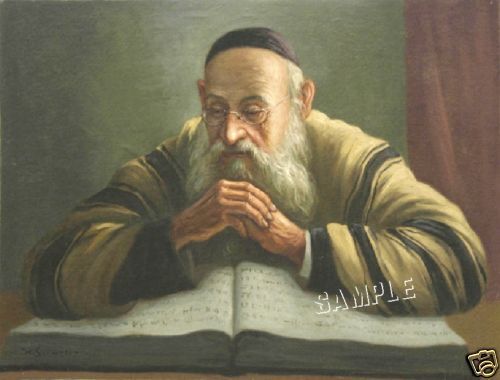The image depicts an illustration of an elderly, scholarly man deeply engrossed in reading a gigantic book resting on a brown table. He has a long, white beard and wears clear glasses, alongside a small, bandana-like hat that suggests a religious affiliation, possibly akin to a yarmulke. The man is dressed in a striped robe of black and yellow. His hands are crossed and positioned in front of his chin, leaning against the open book, which has large, indistinguishable black lettering. The background features a green wall that transitions into a darker red curtain on the right side of the image. The scene is somewhat rough and out of focus, evoking a painted look. Additionally, a watermark and a camera icon with the word “sample” are present in the bottom right corner of the image.